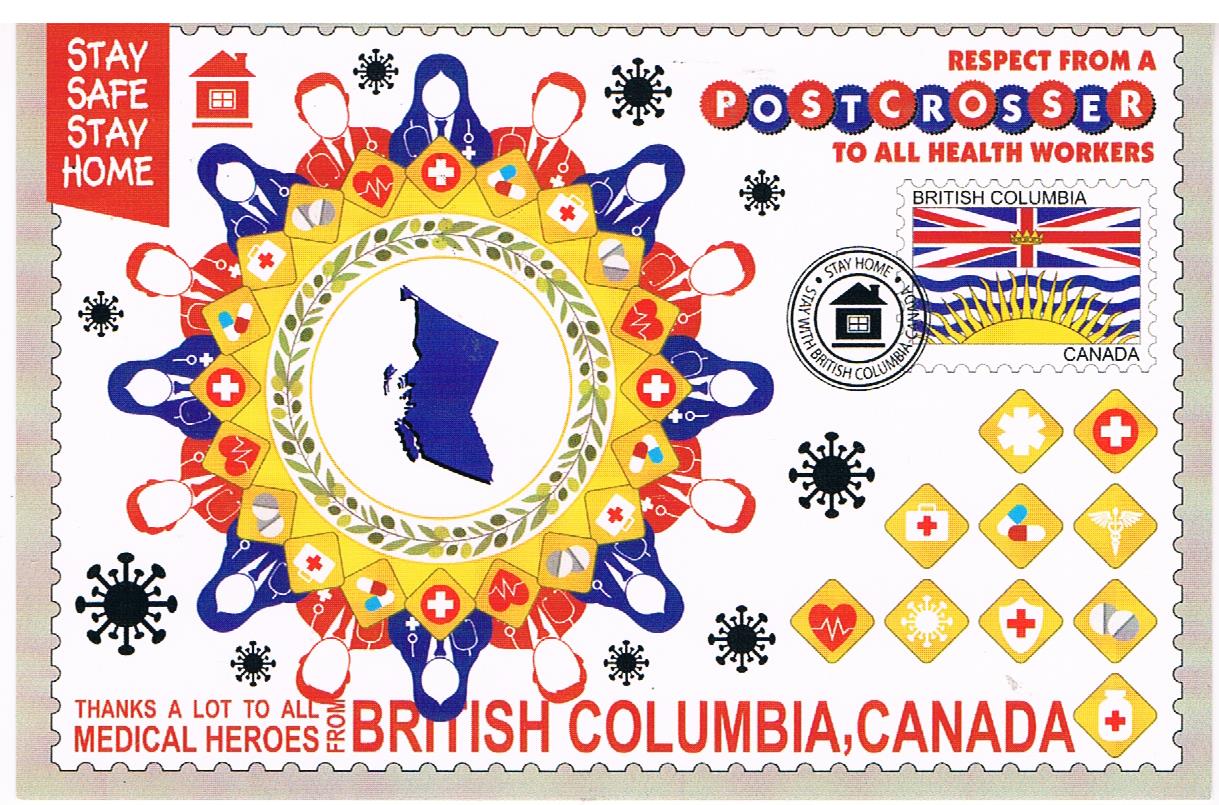This image is a highly detailed, graphic representation of a stamp or postcard, prominently themed around the COVID-19 pandemic. The top left corner features a red banner with the message "Stay Safe, Stay Home" beside a two-dimensional drawing of a small house. At the top right, a red banner reads "Respect from a Post Crosser to All Health Workers," highlighting a tribute to medical professionals. 

The center left of the postcard displays a striking circular emblem with jagged edges, incorporating alternating red and blue images of male and female healthcare workers, both identifiable by the stethoscopes around their necks. Surrounding this circle are various diamond-shaped icons symbolizing healthcare-related items, including a heart, pills, an emergency medical bag, and a medic symbol. Interwoven among these icons are two-dimensional representations of a virus as seen under an electron microscope.

On the right side of the postcard, there's a flag of British Columbia and a phrase that states "Stay Home, Stay with British Columbia Canada," along with another circular emblem featuring a house in its center, emblazoned with the same public health message.

The lower right corner hosts a collection of diamond icons similar to those around the central circle, including EMT stars, medical kits, pills, a Caduceus, an ECG heart, and a shield with a plus sign. The bottom of the postcard carries a heartfelt message in red text: "Thanks a lot to all medical heroes from British Columbia Canada."

Overall, the postcard serves as a detailed visual homage to healthcare workers during the pandemic, mingling regional pride with universal symbols of medical care and safety.